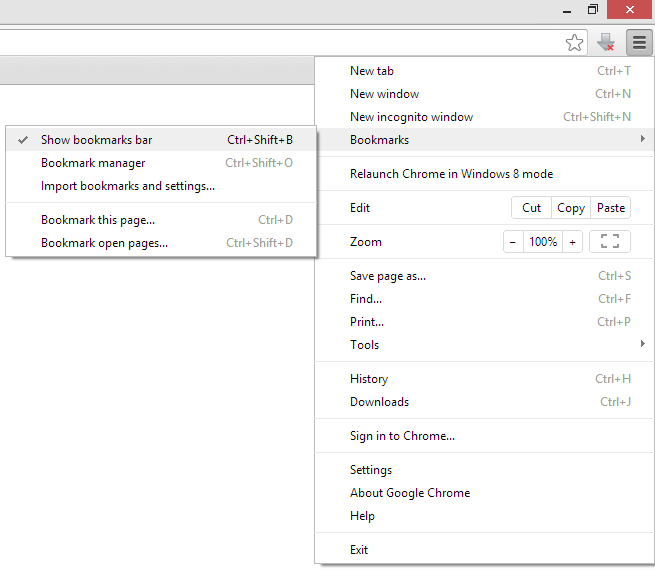The image displays a web browser window with a menu pulled down from the top right corner. The menu showcases various options, including "New tab," "New window," "New incognito window," and "Bookmarks." The "Bookmarks" option has been selected, revealing a secondary, floating menu. Within this floating menu, the "Show bookmarks bar" option is specifically selected, marked by a tick beside it. Other available options in the main menu include "Relaunch Chrome in Windows 8 mode," "Edit," "Zoom," "Save pages," "Find," "Print," "Tools," "History," "Downloads," "Sign in to Chrome," "Settings," "About Google Chrome," "Help," and "Exit." In the floating bookmarks menu, additional options like "Bookmark manager," "Import bookmarks and settings," "Bookmark this page," and "Bookmark open pages" are visible. The rest of the screen shows only a grey caption along the top and a red "X" in the top right corner to close the browser.